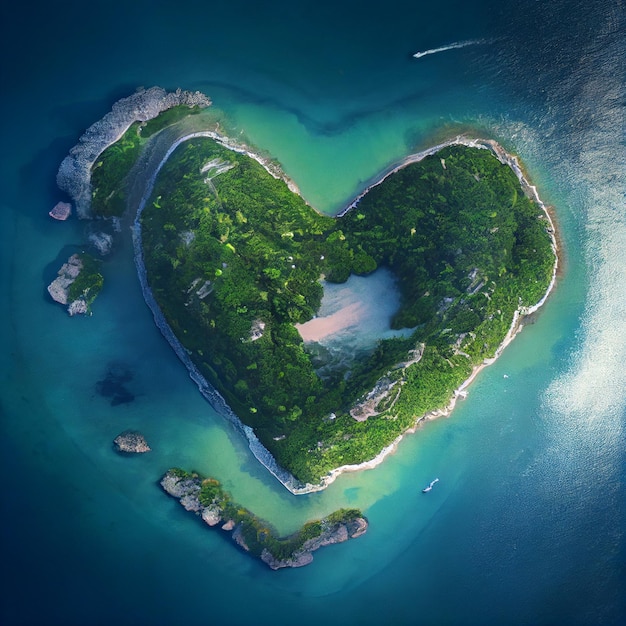This image showcases a digitally created, almost too-perfect heart-shaped island surrounded by a vibrant array of blue ocean hues. The island's perimeter is lush with green vegetation, while the interior features a barer, grayish-white area. A distinctive white border outlines the entire heart, adding to its surreal appearance. The surrounding sea transitions from a light, turquoise blue near the island to a darker blue at the edges of the image. To the top right of the scene, white water trails indicate the approach of a boat, possibly a yacht. Additionally, there are several rocky outcrops nearby, including a landmass to the top left, another to the middle left, and a V-shaped spit of land at the bottom point of the heart. The entire setup exudes a typical tropical island charm with an artistic twist.